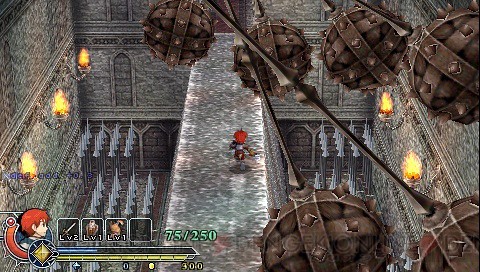This image is a screenshot from a video game. In the bottom left corner, there is a character with orange hair, appearing to navigate through the game. Adjacent to the character, there is an inventory consisting of four squares: one containing a sword, another square is blank, and the remaining two contain undefined items. In addition, there is a counter displaying "75 out of 250."

In the center of the image, a stone bridge is prominently featured, with the orange-haired character crossing it and seemingly equipped with a sword. On both sides of the bridge are perilous gaps filled with gray spikes, posing a threat to anyone who might fall. Suspended from the ceiling are brown lines, each ending with large, spiked spherical objects. The character must skillfully traverse the bridge while avoiding these hazardous obstacles.